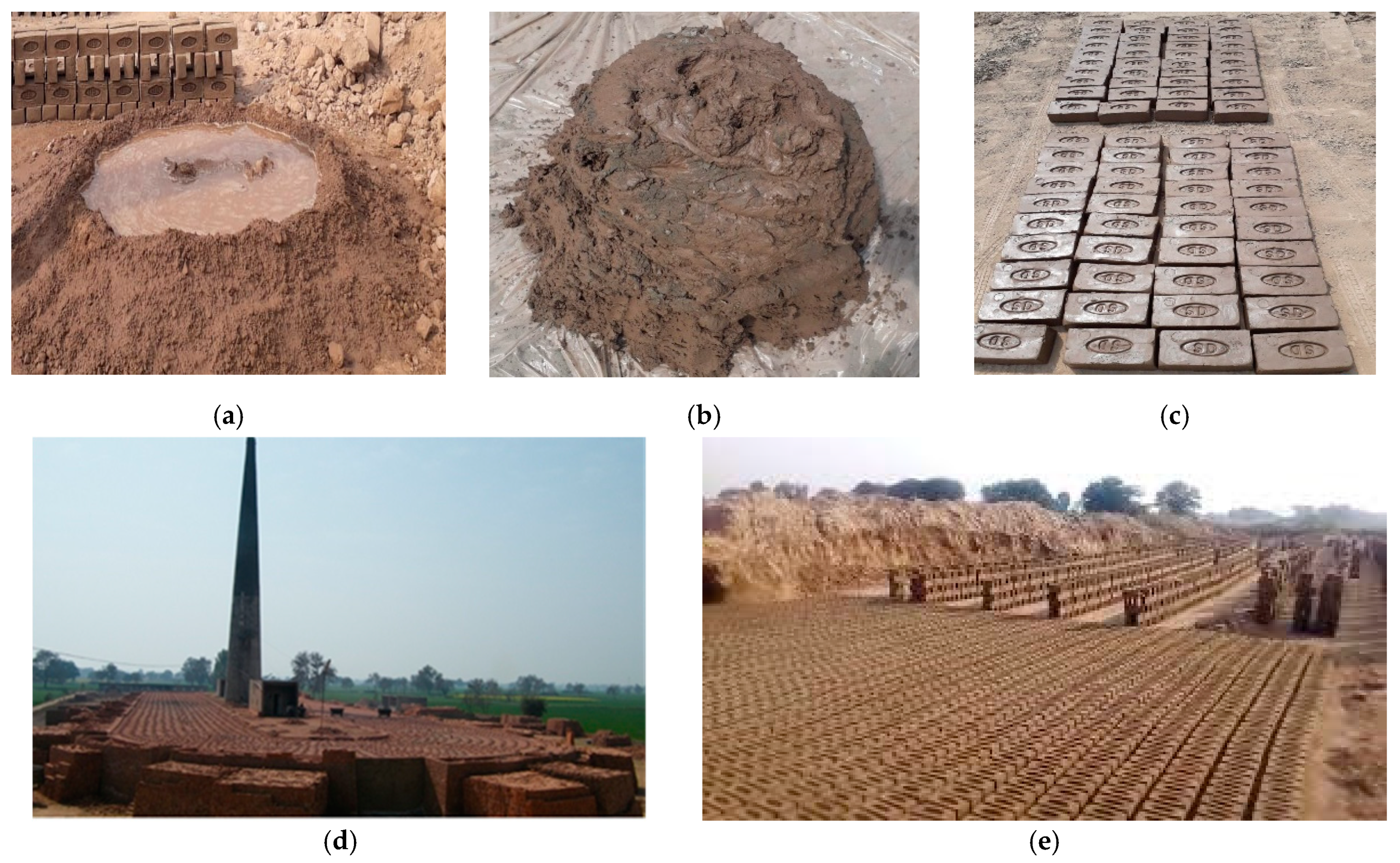The image consists of five separate photographs labeled A through E. Three images (A, B, and C) are arranged horizontally at the top, while two images (D and E) are placed horizontally at the bottom. 

In image A, there's a hollowed-out mound of dirt with water pooled in its center, appearing brown and framed by bricks in the background. Image B showcases a pile of brown and gray mud situated on a white or clear plastic tarp, suggesting early stages of material preparation. Image C depicts rows of thin, brown ceramic tiles or bricks, each possibly featuring a round seal in the middle, organized into two groups of four rows that extend into the backdrop.

Moving to the bottom row, image D presents a landscape with green grass, trees, and a light blue sky in the background. In the foreground and mid-ground, there's a large cylindrical structure, possibly a tower or chimney, amidst stacks of mud bricks. Lastly, image E displays a large area, possibly half an acre or more, filled with stacks and rows of these bricks or tiles, with a prominent mud wall in the background. The repetitive arrangement and the outdoor setting hint at a large-scale production or storage site.